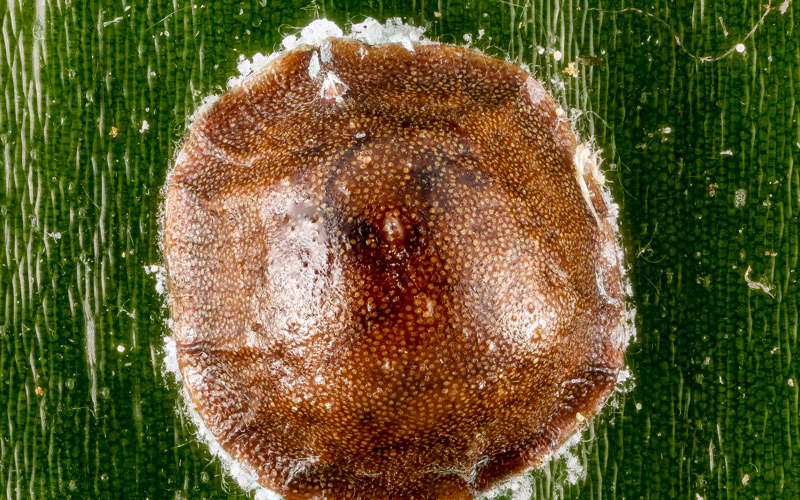This highly detailed close-up image, taken from an overhead perspective, depicts a mysterious, roughly circular brown object occupying the center of the frame. The object, possibly a living organism or a natural formation like a mushroom, has a somewhat domed, shiny texture reminiscent of a young frog or an unopened bud. Surrounding the brown entity is a white, fluffy substance, resembling cotton or fabric strands, adding to its enigmatic appearance. The background is a vibrant hunter green, possibly resembling tall grasses or a large leaf with visible striations and cells, adding texture to the scene. The brown object, described as having the color of toast, takes up most of the horizontal rectangle, with about a quarter of the frame on each side revealing the verdant background. Despite varied interpretations, ranging from a tadpole or spore to an object caught on fabric, the well-lit image's complexity encourages curiosity and closer examination.